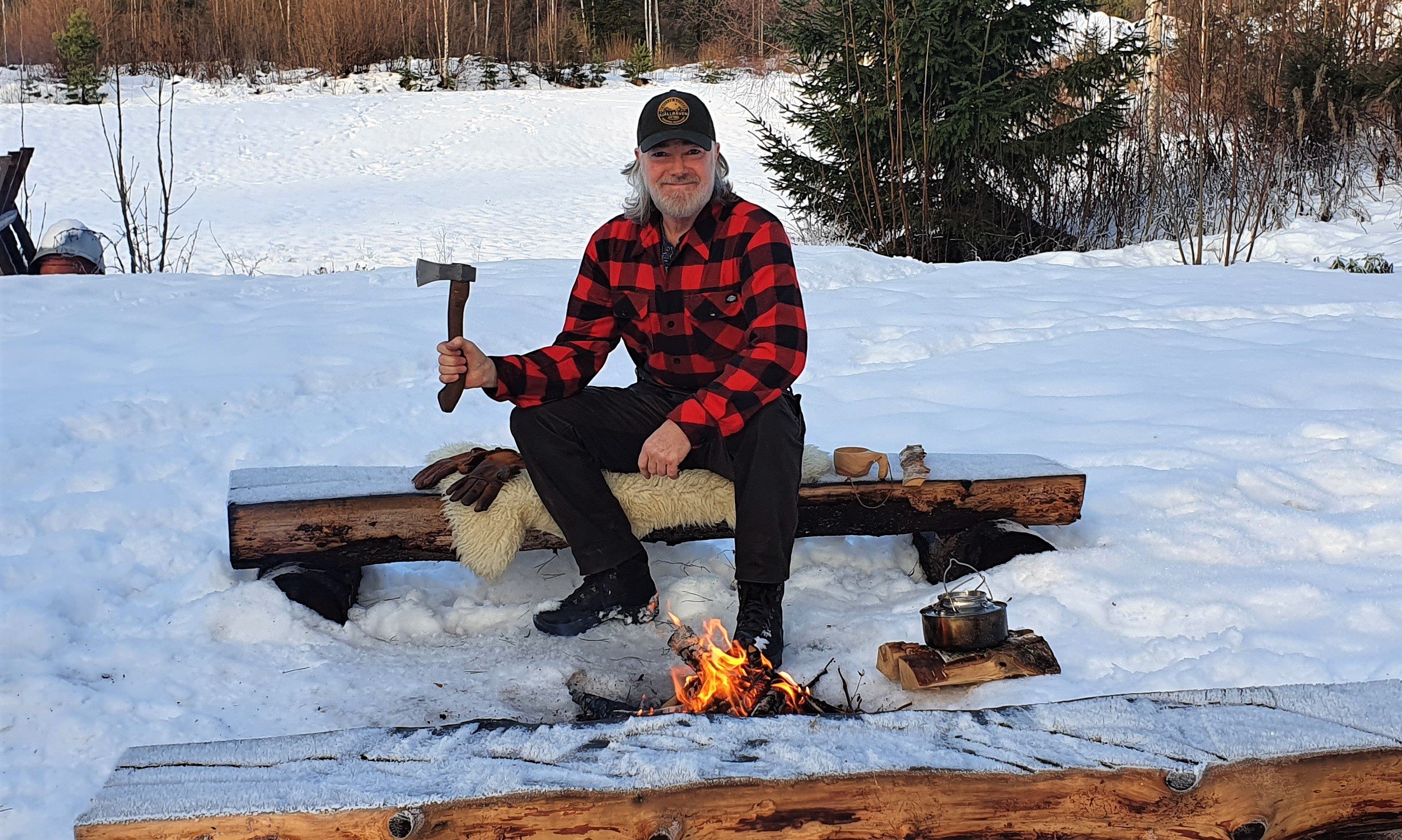In a serene winter landscape, an older man, donned in a red and black buffalo check flannel shirt, black pants, and sturdy hiking boots, sits comfortably on a log bench cushioned with a sheepskin. His gray hair and full gray beard add to his rugged, lumberjack-like appearance. A black ball cap adorned with an orange insignia crowns his head. He holds a small axe proudly in his right hand, as he smiles warmly at the camera. Beside him, on the log, lay a pair of work gloves and a small camp cup, presumably for his hot tea or coffee. In front of him, an open campfire crackles, with a cook pot perched on split logs nearby. The surrounding snow-covered ground and distant fir trees enhance the tranquil, wooded setting. The man appears to be enjoying his peaceful moment in nature, perhaps warming up in the cold and savoring the rustic charm of his snowy campsite.